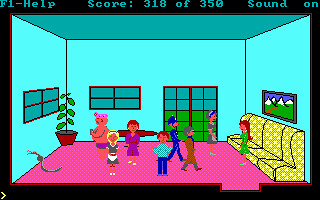This pixelated screenshot from an old-school video game captures a cozy room inside a house. The room features a reddish floor and, along the right-side wall, a couch where a person in a green dress is seated. Above the couch, there's a painting or sign adorning the wall, adding a touch of decor to the space. The back wall boasts sliding windows with four-pane designs, letting in virtual light. In the middle of the frame, several characters gather, bringing the room to life with their presence.